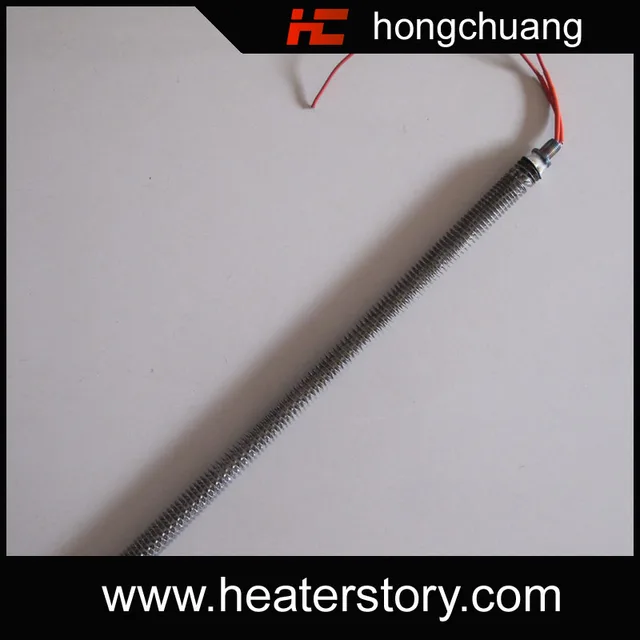This is a detailed, close-up image of a mechanical component, possibly a heating element, with significant magnification. The object, resembling a long, thin metal rod with deep threads or barbs, is positioned diagonally and leans slightly towards the bottom right of the image. It features a prominent spring-like structure near its middle and has two red wires extending from its top, curving outward before being cut off by the image border. The surface on which the component rests is plain white, creating a clear shadow that adds depth and confirms its placement on a physical surface. The colors visible in the image include red, black, white, off-white, gray, and silver. The top of the image displays the manufacturer’s name, "Hong Chuang," in white text within a black bar, accompanied by a stylized red "HC" logo. Below, another black bar runs across the bottom, containing the website "www.heaterstory.com" in bold, white sans-serif text. This product is likely intended for home improvement purposes and could be typically found in a hardware store.